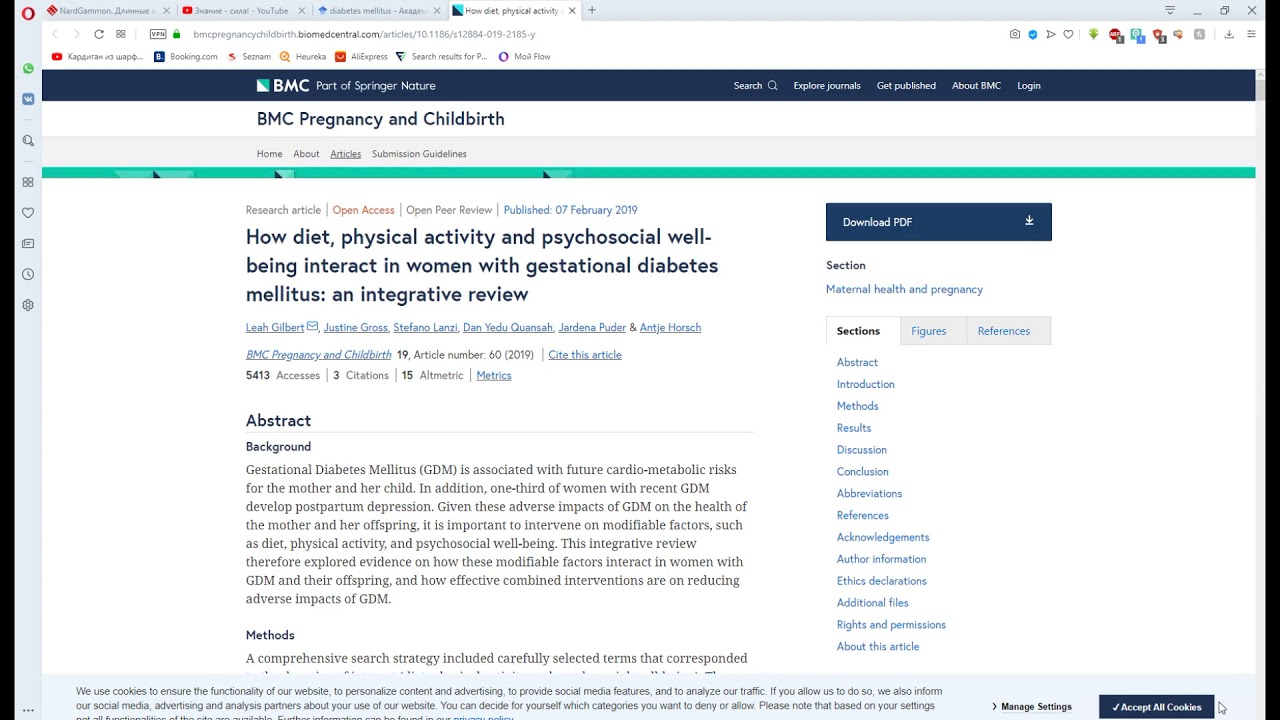The screenshot displays a web browser window with four open tabs, although the specific titles of these tabs are not legible. In the bookmarks bar, identifiable bookmarks include Booking.com and a YouTube icon, though the rest are unreadable. Under the bookmarks, text reads, "BMC, part of Springer Nature." There is a search function next to options labeled "Explore Journals," "Get Published," "About BMC," and "Login."

Beneath this, the page heading reads "BMC, Pregnancy and Childbirth," followed by navigation links that include "Home," "About," "Article," and "Submission Guidelines." Further down is a teal-colored horizontal stripe extending across the screen, below which the text indicates the section is "Research Article" with tags "Open Access" and "Open Peer Review." The article was published on 07 February 2019, titled "How Diet, Physical Activity, and Psychosocial Wellbeing Interact in Women with Gestational Diabetes Mellitus: An Integrated Review."